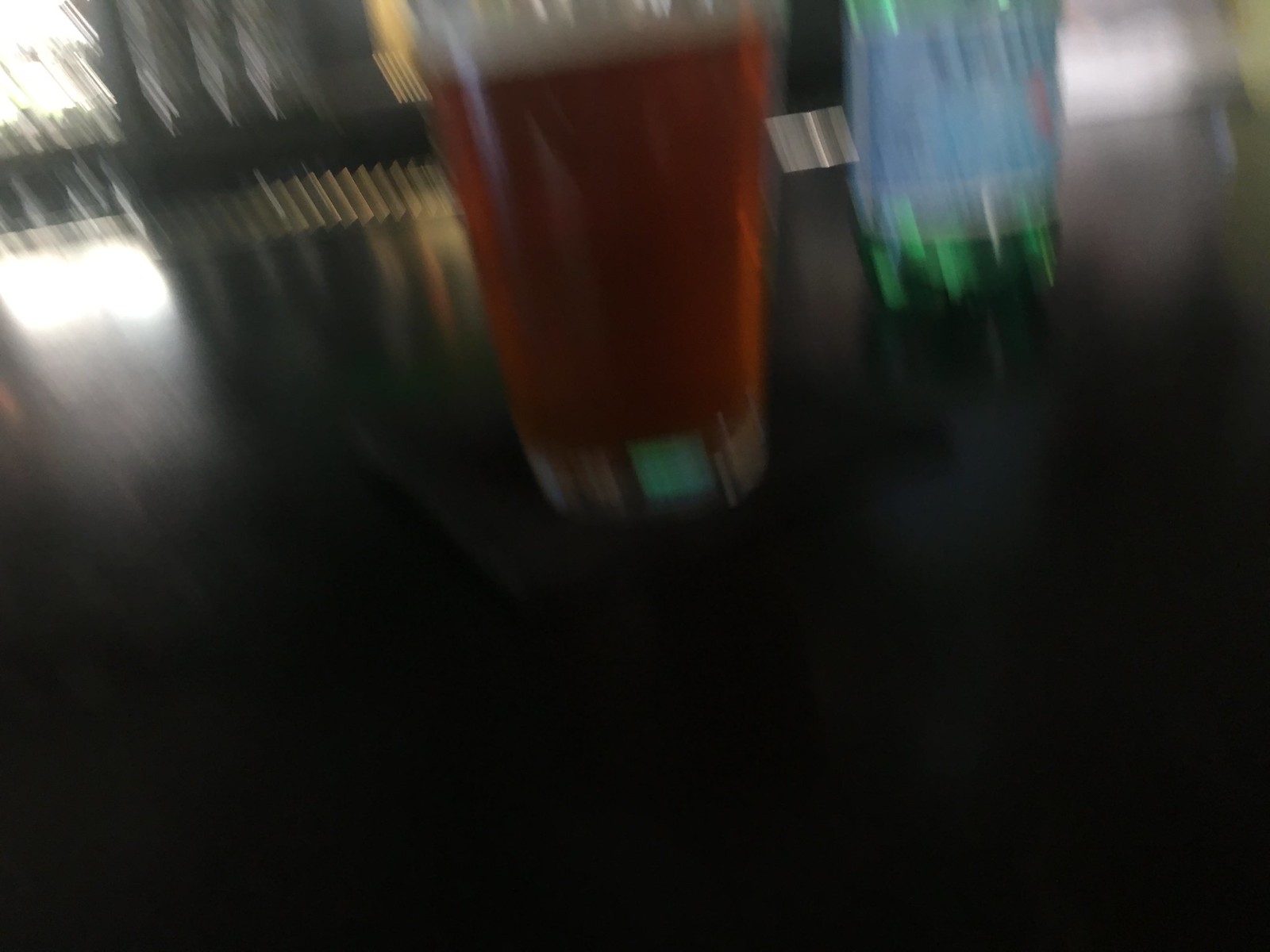The photo is extremely blurry and of very low quality, giving it a fuzzy appearance that suggests the camera was moving when the picture was taken. The main focus seems to be on a dark wooden counter, illuminated by a light source from a window in the back left corner, which is partially obscured by white shades. On the counter, there is a tall, clear pint glass filled with a golden-brown beer that has a foamy head, resting on a black napkin or coaster. Adjacent to the beer glass and slightly set back is a green glass bottle with a white label that is partly cut off, making the label unreadable. The label appears to have light blue and white stripes with some darker blue writing and a bit of red detail. This bottle might be a sparkling or mineral water. Despite the extreme blurriness, it seems like the setting could be a bar or a table, as indicated by the lights visible in the background.